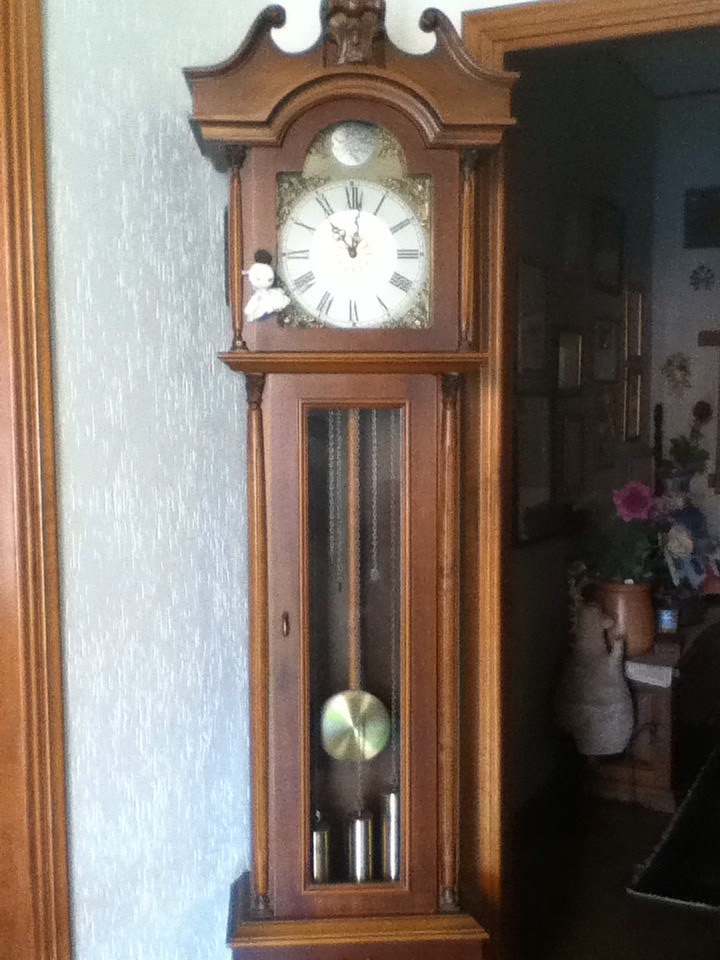In the image, a large wooden grandfather clock is prominently displayed against an indoor wall. The wall, adorned with a textured gray finish, possibly from wallpaper or a specialized treatment, contrasts elegantly with the dark wood trim that frames it. To the side, there is a small glimpse into an adjacent room, revealing a flower pot and a few pictures hanging on the wall. The grandfather clock itself is crafted from rich, dark wood, giving it a stately presence. Its face is white, detailed with black Roman numerals and black hands, standing out in clear contrast. The image is void of any text, focusing purely on the intricate details and atmosphere of the scene.